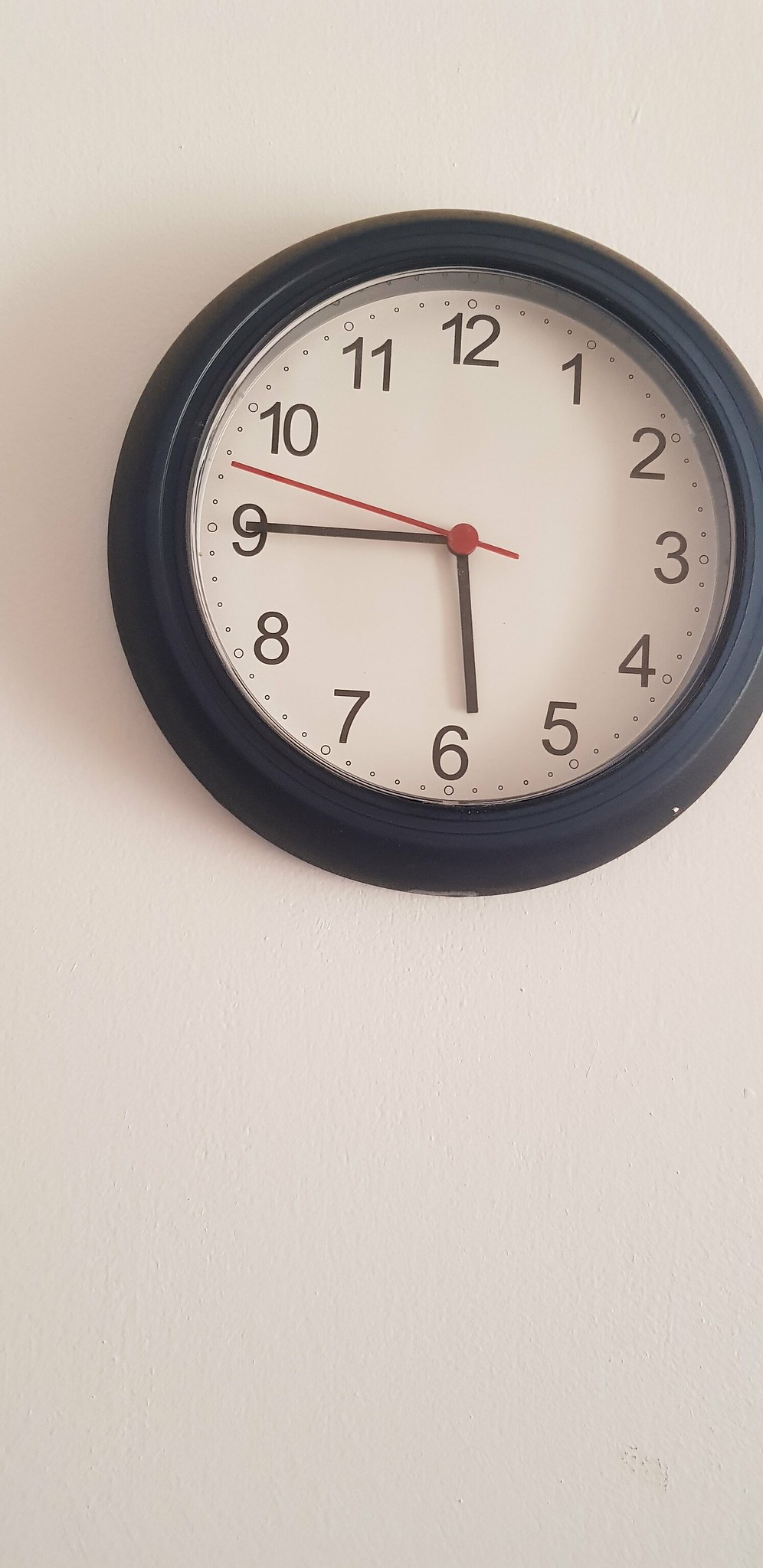A simple yet classic wall clock is perched against a white wall. This circular timepiece features a minimalist design with black sides and a plain, unassuming white face. The numerals, ranging from 1 to 12, are rendered in a traditional Times New Roman font, also in black. Both the hour and minute hands are black, while the second hand stands out in a bold red, adding a touch of color to the monochrome palette. The clock's straightforward design and complete numbering make it a functional and unobtrusive addition to any setting.